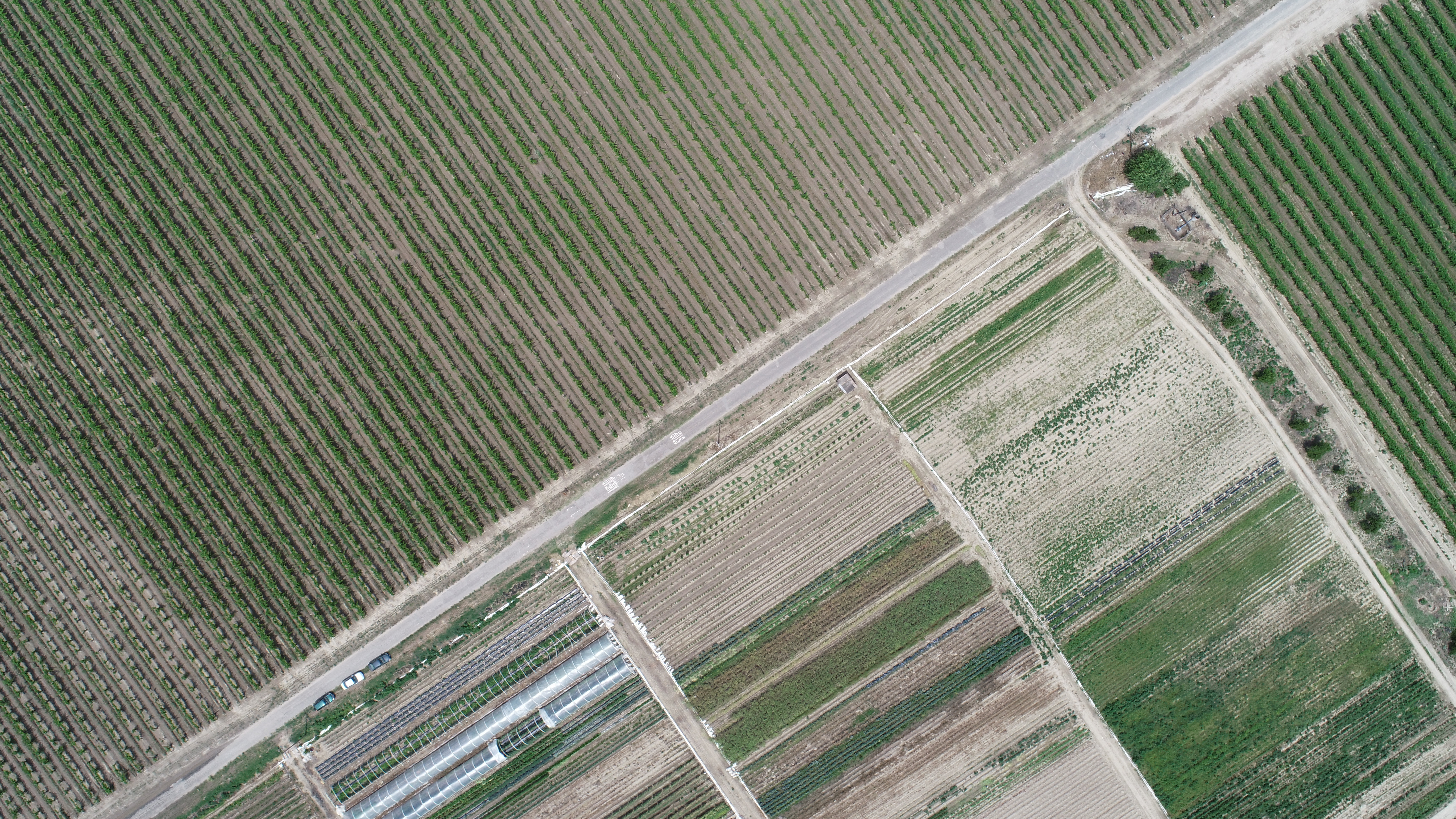This highly detailed and clear aerial photograph, likely taken by a drone, captures a vast expanse of agricultural farmland bathed in bright, natural daylight. The central focus of the image is a small, somewhat narrow two-lane road that stretches diagonally from the bottom left to the top right of the photograph. Along this road are vehicles parked on the dirt shoulder in the bottom left corner, and within the road itself, the word "STOP" is painted in both directions.

On the left side of the road, the farmland consists of numerous neatly arranged rows of green crops, all running perpendicular to the road. To the right of the road, small dirt paths branch off, interspersed with more green crop fields, whose rows also run perpendicular to the main road. Additionally, there are sections of open dirt fields, and scattered trees dot the landscape. In the upper right corner, a few houses or housing units can be seen, along with what appears to be a greenhouse structure. The entire scene is depicted in vivid color, showcasing a variety of green hues from the crops and the earth tones of the dirt paths and fields.